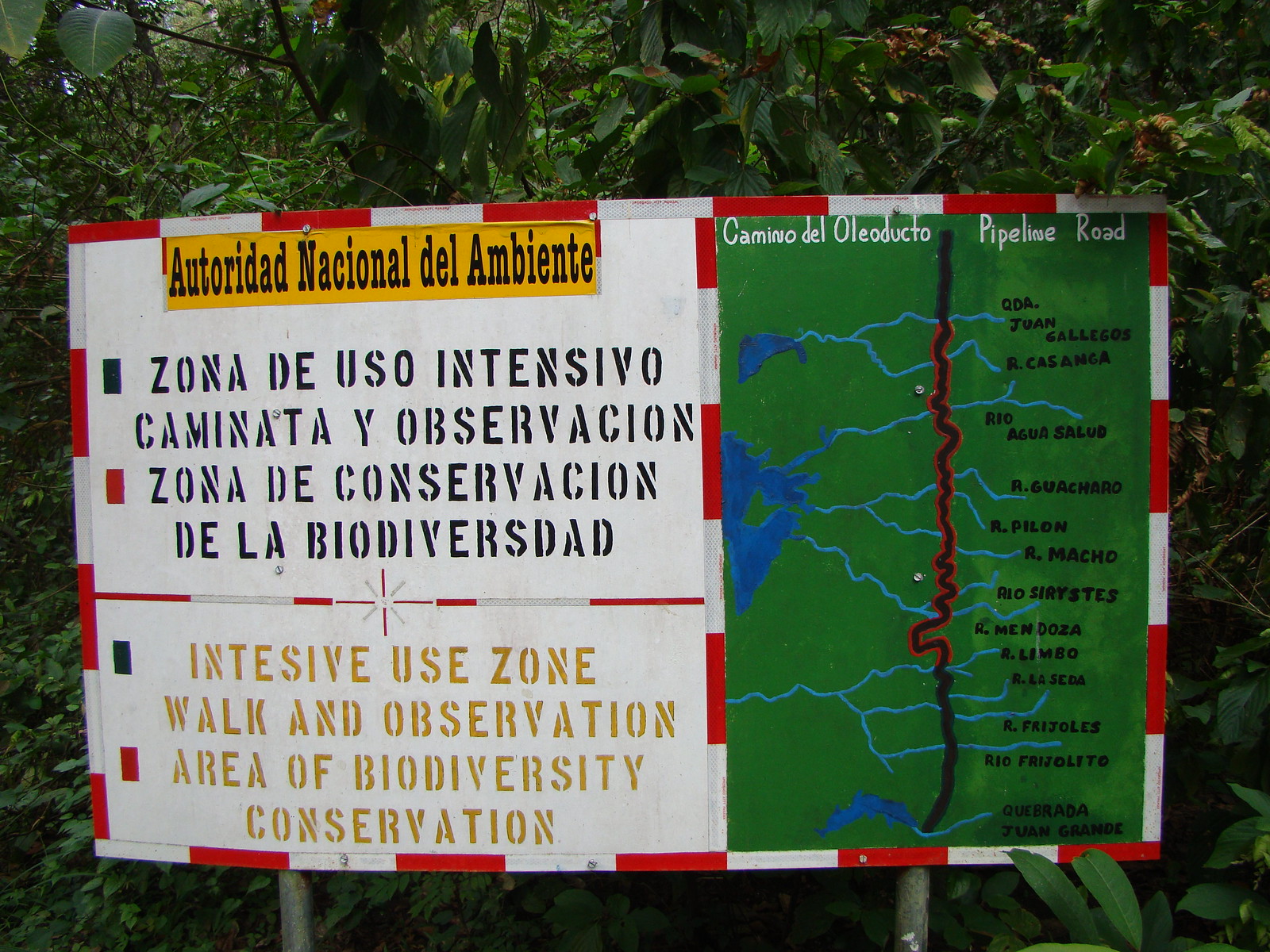This image depicts a rectangular sign standing amidst dense forest foliage. The sign, bordered by a red and white stripe, features three sections. The top left corner has a yellow banner with Spanish text, "Autoridad Nacional del Ambiente" followed by "Zona de Uso Intensivo, Caminada y Observación, Zona de Conservación de la Biodiversidad" written in black letters. Directly below, in dark yellow letters, it reads in English: "Intensive Use Zone, Walk-in Observation Area of Biodiversity Conservation." The right side of the sign displays a roadmap with a blue and red line indicating a pipeline route traversing through the forest and marking points labeled "Rio," "Agua," "Salud," "Rio Frigio Leto," and others. The lush green backdrop with trees and bushes engulfs the sign, blending it seamlessly into its natural surroundings.